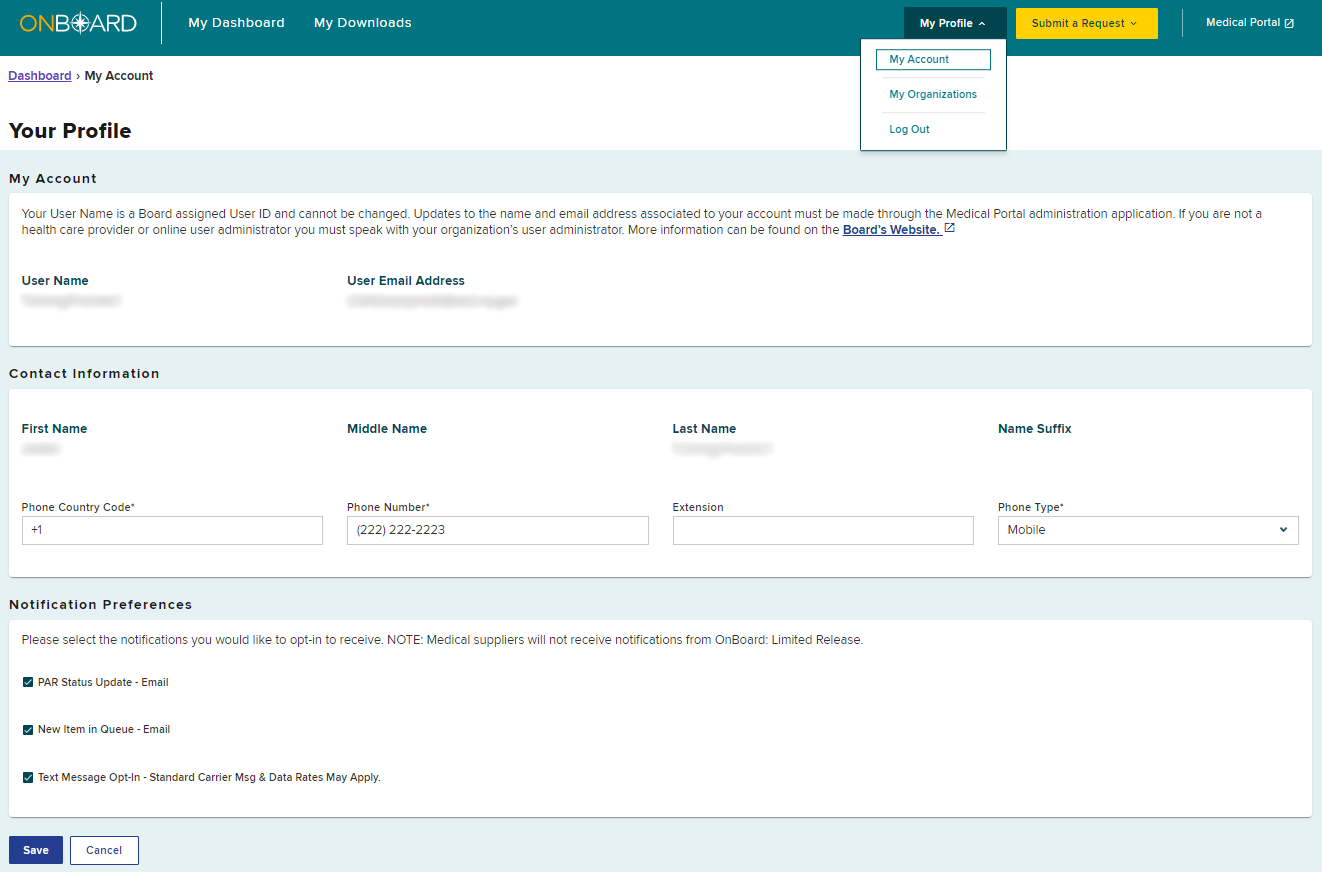This screenshot depicts a user navigating through their account settings on a medical portal website. At the top of the interface, there are several navigation tabs labeled "On Board," "My Dashboard," "My Downloads," and "My Profile." A dropdown arrow has been clicked, revealing options such as "My Account" (which is selected), "My Organizations," "Log Out," "Submit a Request," "Medical Portal," "Dashboard," and another instance of "My Account."

The page contains instructions that the username, assigned by the board, cannot be changed. Updates to the name and email address must be made through the Medical Portal Administration application. Non-healthcare providers or online user administrators are directed to consult their organization's user administrator. Additional details are available on the board's website.

Personal information fields such as the user's username, email address, first name, and last name are blurred out. The "Medical name" field is left blank. The user’s phone information includes a country code of "+1" and a phone number formatted as "222-222-2223," with the extension field blank. The phone type is specified as "mobile."

Under "Notification Preferences," users are prompted to select notifications they wish to receive, noting that medical suppliers will not get notifications from the limited release of the On Board system. Options include receiving PAR status updates via email and new items in the queue also via email. There is also an option to opt-in for text message notifications, with a note that standard carrier message and data rates may apply.

Buttons for "Save" and "Cancel" are located at the bottom of the page.